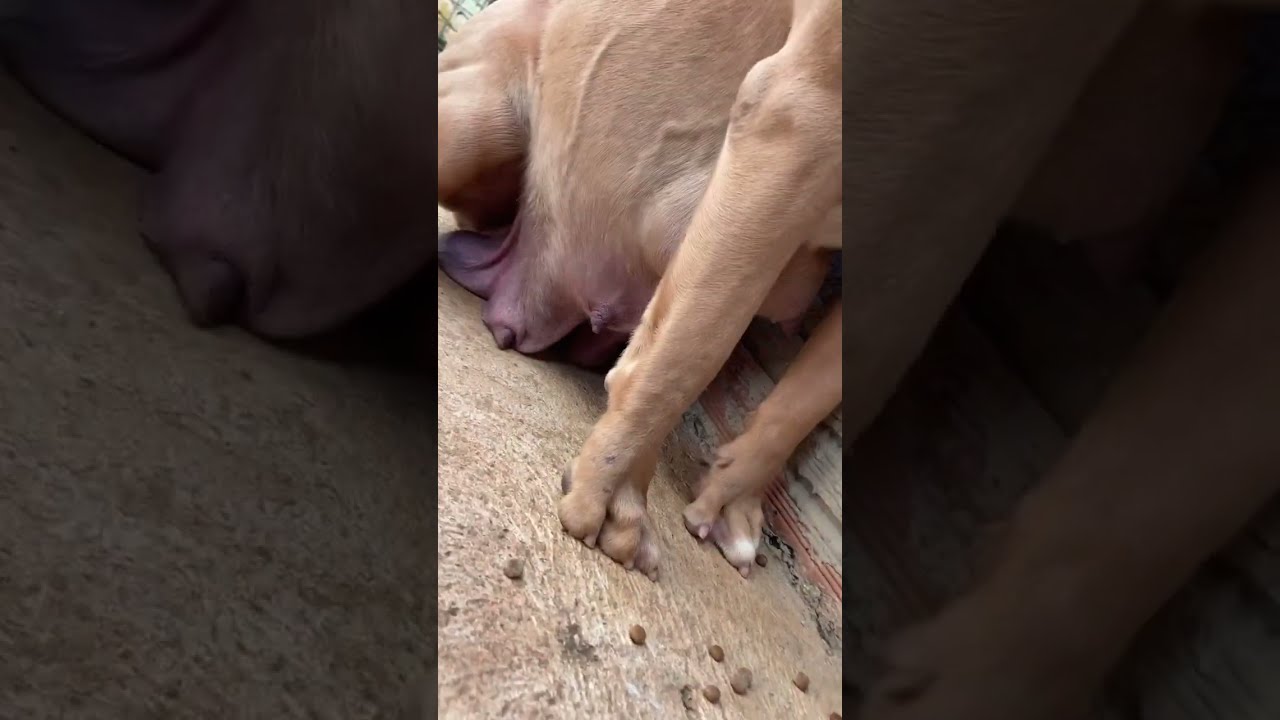The image is a photograph of the lower part of a light brown, pregnant, or nursing female dog positioned centrally against a rough, raw wood floor that resembles plywood. The painting on the wall behind the dog is chipped and used to be red. The sides of the image are obscured by dark, blurred overlays that take up about a third of the image on both the left and right, drawing attention to the dog at the center. The dog is depicted with her front legs extending toward the ground, showcasing distinct white tips on her toes and pink toenails. The dog's back leg appears to be leaning or squatting. Dominating the central focus are her swollen, distended breasts, exhibiting some discoloration with purple and red hues, indicating she may have recently been nursing. Scattered in front of her front paws are small, circular pieces of brown dog food.